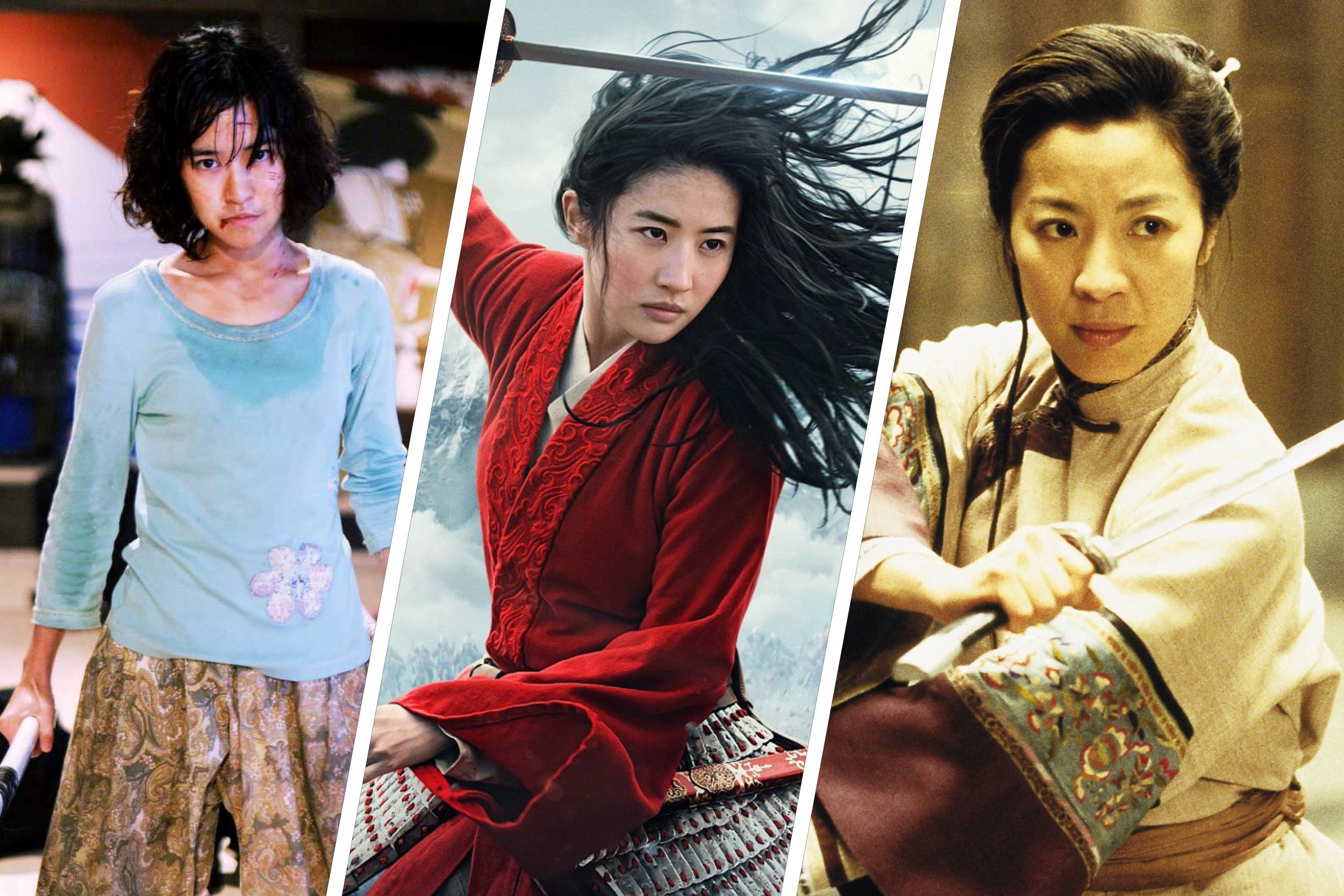This image depicts three significant phases of Michelle Yao's career through a trio of photographs, each capturing her in different characters and moments. On the left, a young Michelle Yao with short, dark hair and an intense expression wears a blue long-sleeved shirt with visible sweat at the rim and a flower design, paired with a gold paisley skirt. She has a bloodied lip and clenches a weapon in her right fist. The central image shows Yao as a warrior from Mulan, clad in a red velvet jacket over white garments and a metallic, armored skirt. Her black hair flows as she raises a sword diagonally above her head, prepared for combat against a mountainous backdrop. The far-right photograph features an older Michelle Yao dressed in an intricately embroidered white kimono with teal trim and a brown belt, her hair styled in a bun. She holds a sword angled back past her body, ready and focused, embodying a poised and seasoned warrior. Each image distinctly showcases Michelle Yao's dynamic and powerful on-screen presence.